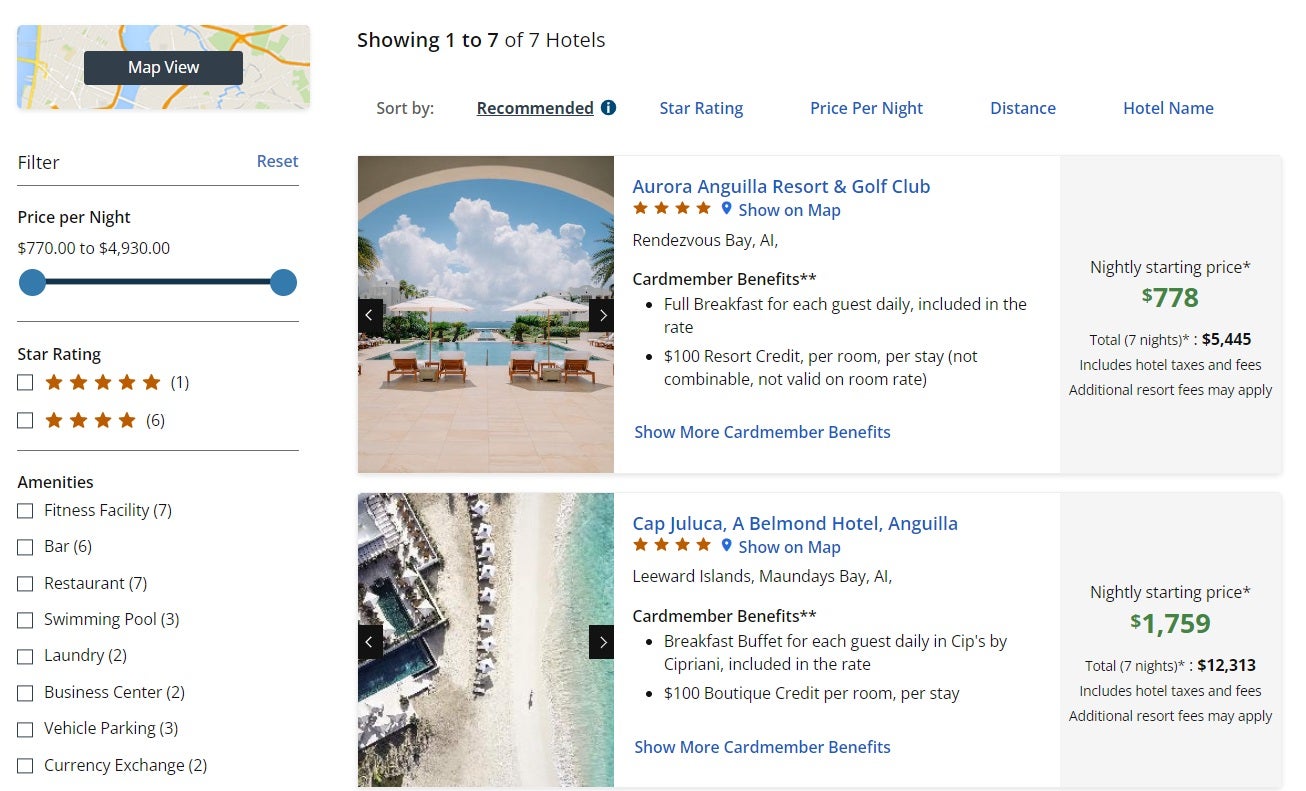The image is a screenshot of a hotel booking interface. On the left side, various options and filters are displayed for selecting accommodations. At the top, it reads "Map View," followed by "Filter Reset." The price range for a night's stay is listed as $770 to $4,930. The next section, "Star Rating," features five stars, with one option selected, and four stars with a note indicating six hotels available.

A black horizontal line separates this section from the "Amenities" category below. Each amenity has a checkbox to the left, and the following amenities are listed from top to bottom: Fitness Facility (7), Bar (6), Restaurant (7), Swimming Pool (3), Laundry (2), Business Center (2), Vehicle Parking (3), and Currency Exchange (2).

On the right side, it states "Showing 1 to 7 of 7 hotels." Beneath this, sorting options are provided, including: "Recommended," "Star Rating," "Price per Night," "Distance," and "Hotel Name." The example hotel shown is "Aurora, Anguilla Resort and Golf Club."